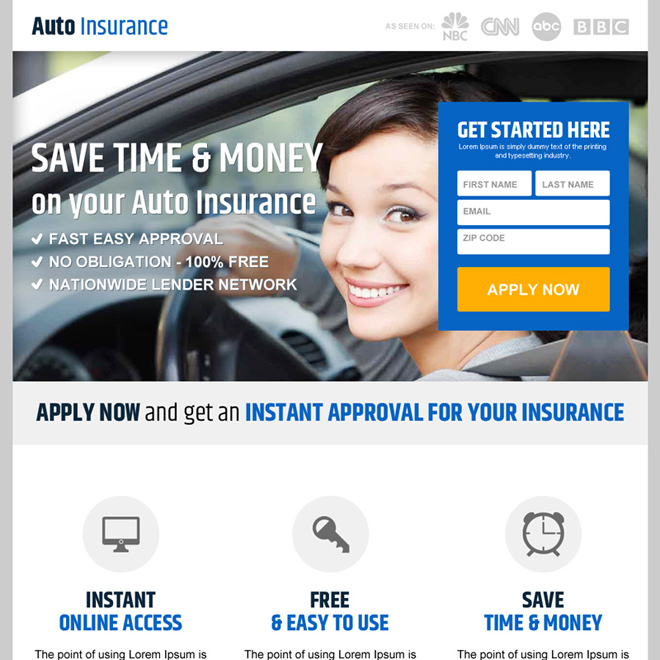Screenshot of an Insurance Website:

The screenshot depicts an insurance website, clearly identified by the header at the top left that reads "Auto Insurance." The logo itself features the words "Auto" in black text and "Insurance" in blue text.

In the top right corner, there are several logos that appear to be grayed out. These include recognizable logos such as CNN, HBO, and BBC, along with two other indistinguishable ones.

Directly beneath the logos and the main title is a prominent splash image. The image features a large, bold statement in white text: "Save Time and Money on Your Auto Insurance." On the left side of this image, there is a list, or bullet point section, highlighted with check marks. The list includes the following points:
- Fast, easy approval
- No obligation
- 100% free
- Nationwide lender network

On the right side of the same splash image, there is a "Get Started Here" section. This section contains fields where users can input their first name, last name, email, and zip code. Beneath these input fields is an orange "Apply Now" button.

Below this button, additional information is provided, stating:
- Instant online access
- Free and easy to use
- Save time and money